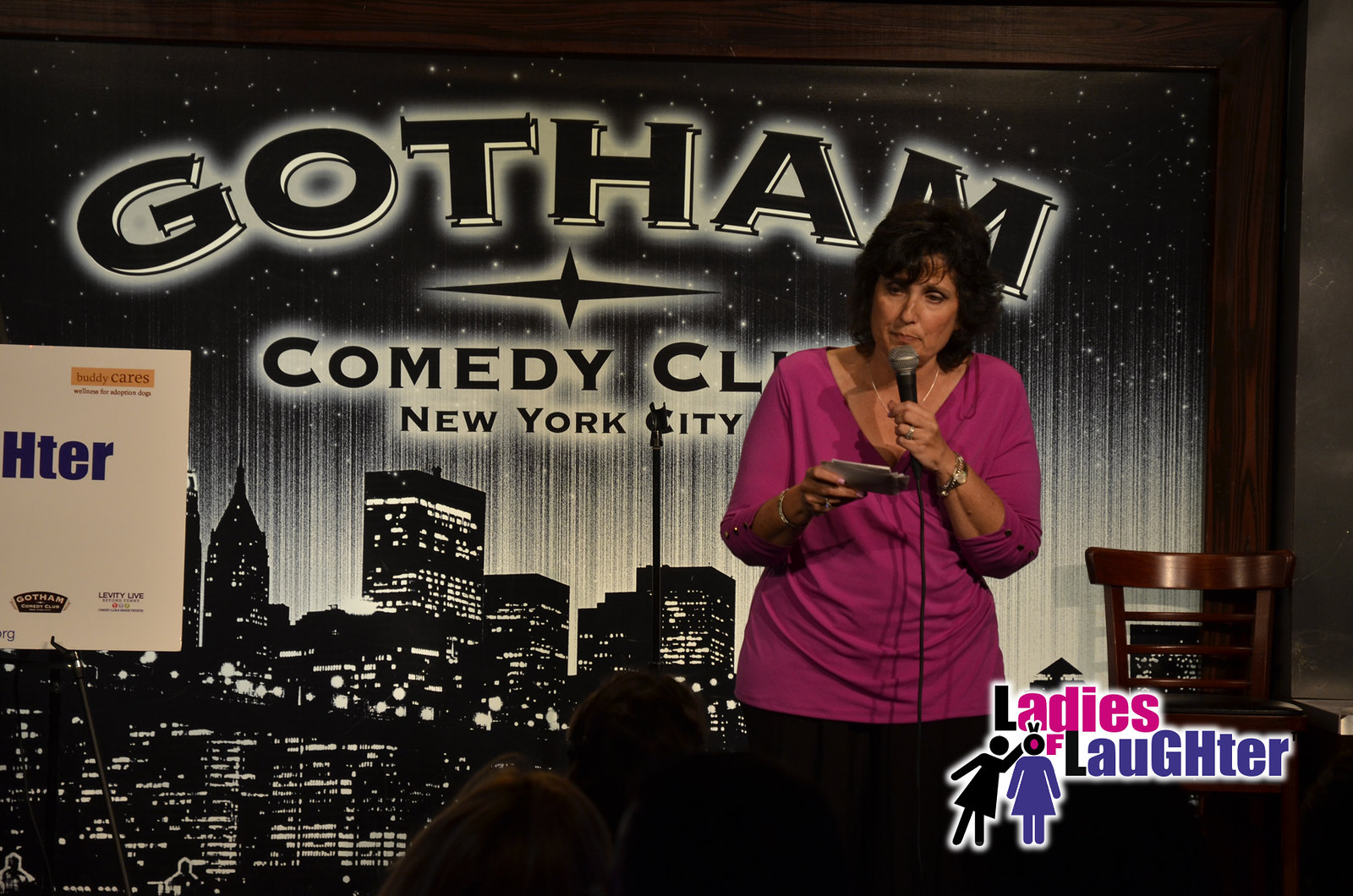The photograph captures a female comedian on stage at the Gotham Comedy Club in New York City. She is dressed in a long-sleeved, v-neck shirt in a pinky fuchsia maroon color, with her sleeves pushed up to her elbows. She is holding a microphone close to her mouth with her left hand, which also wears a wristband, while her right hand holds cards likely containing her jokes, and sports a bracelet. She appears to be interacting with the audience, although the audience is not visible in the image.

Behind her, a wooden chair is placed slightly to her left, adding to the intimate atmosphere of the club. The backdrop prominently displays the Gotham Comedy Club logo along with monochrome images of buildings, solidifying the New York City vibe.

In the bottom right corner of the image, there is a colorful logo in pink, black, and blue that reads "Ladies of Laughter," featuring two stick figure icons. This suggests that the event is a comedy show exclusively showcasing female comedians. To the far left of the frame, partially covering the Gotham Comedy Club backdrop, is a white poster with blue text and yellow and black logos, though only half of it is visible due to the crop of the photograph. A microphone stand without the microphone can also be seen, positioned in front of her.